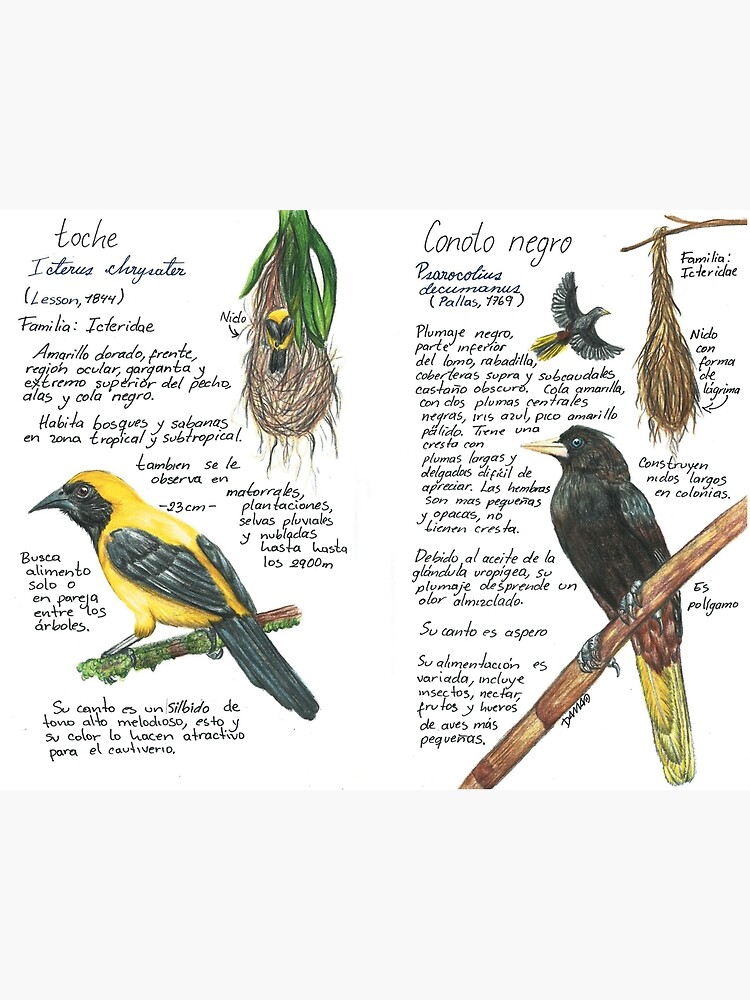This detailed botanical illustration comprises two different bird species, each displayed with significant ornithological features and text descriptions in Spanish. On the left side, the page is labeled "Toche," identifying a bird from the Icteridae family. This yellow bird features black wings, a black tail, and a black face. Adjacent to the bird's depiction is its nest, which hangs from a branch adorned with green leaves. Below this image, the vibrant Toche is seen perched on a twig with green accents, gazing to the left.

The right side, labeled "Conoto Negro," portrays another bird from the same family. This bird is primarily black but with distinct yellow undersides on its tail. The top illustration of the Conoto Negro shows it in flight, while the bottom image shows it perched on a dark stick, also facing left. This side includes an analogous hanging nest entwined with a branch. The detailed Spanish text includes descriptions of each bird's habitat, song, and behaviors, adding scientific context to the visual artwork.